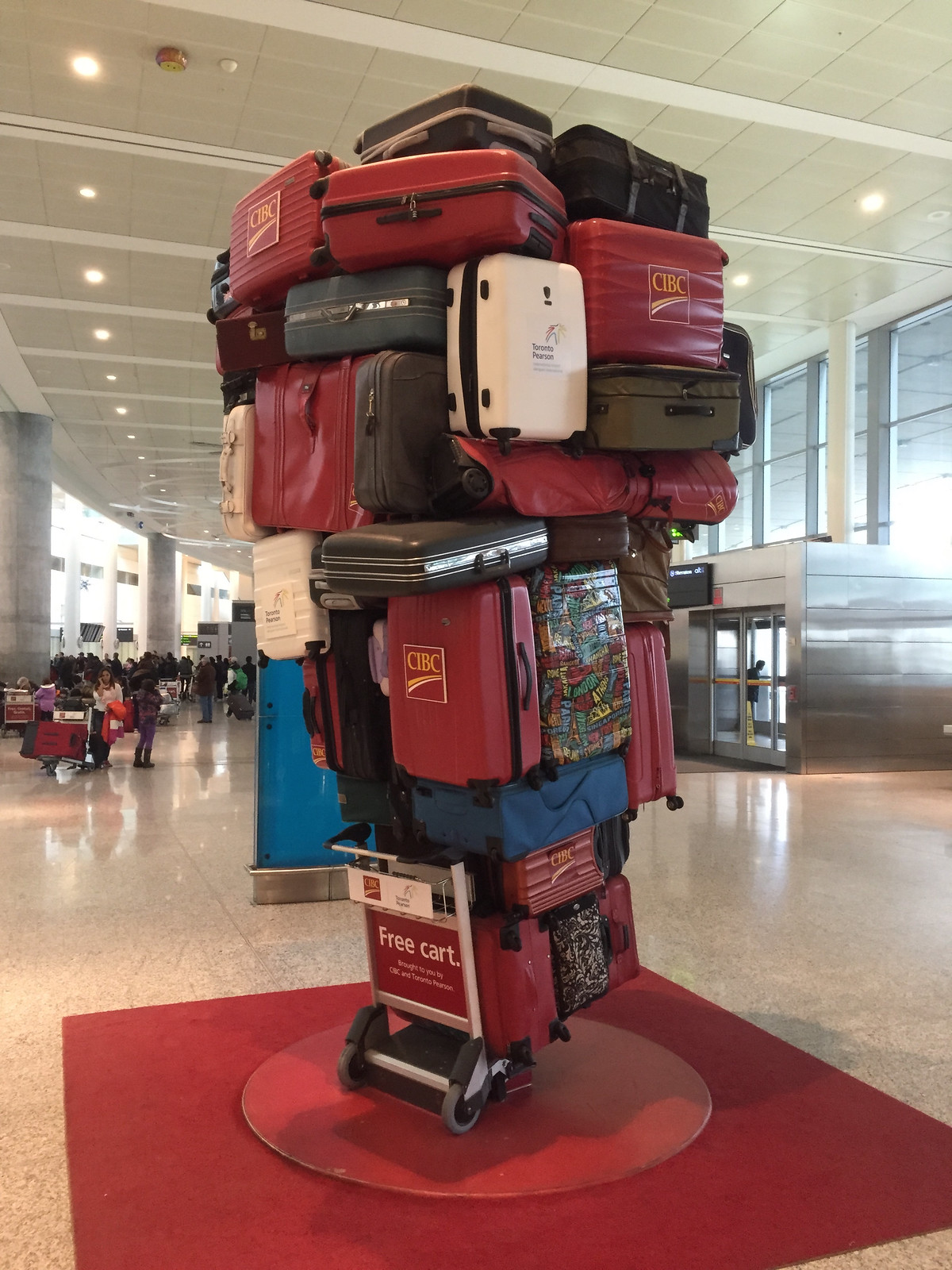This photograph captures a vibrant and intriguing scene inside an airport, featuring a towering sculpture made of luggage. In the foreground, situated on a red square rug, there's a silver airport cart with a banner that reads "Free Cart." However, this is no ordinary cart; it is humorously stacked with approximately 25 to 30 pieces of luggage, creating an almost whimsical artistic display. The suitcases, in a variety of colors with a notable number in red, alongside blues, blacks, browns, and whites, are piled so high they nearly touch the ceiling. In the background, on the right side of the image, you can see the airport entrance with sliding doors and a metal gate. To the left, a corridor flanked by tall white cement columns leads off into the distance. Beyond the sculpture, one can observe passengers pulling their luggage, adding to the bustling atmosphere of the terminal. This playful, eye-catching installation juxtaposes the practical with the artistic, blending seamlessly into the everyday hustle of airport life.